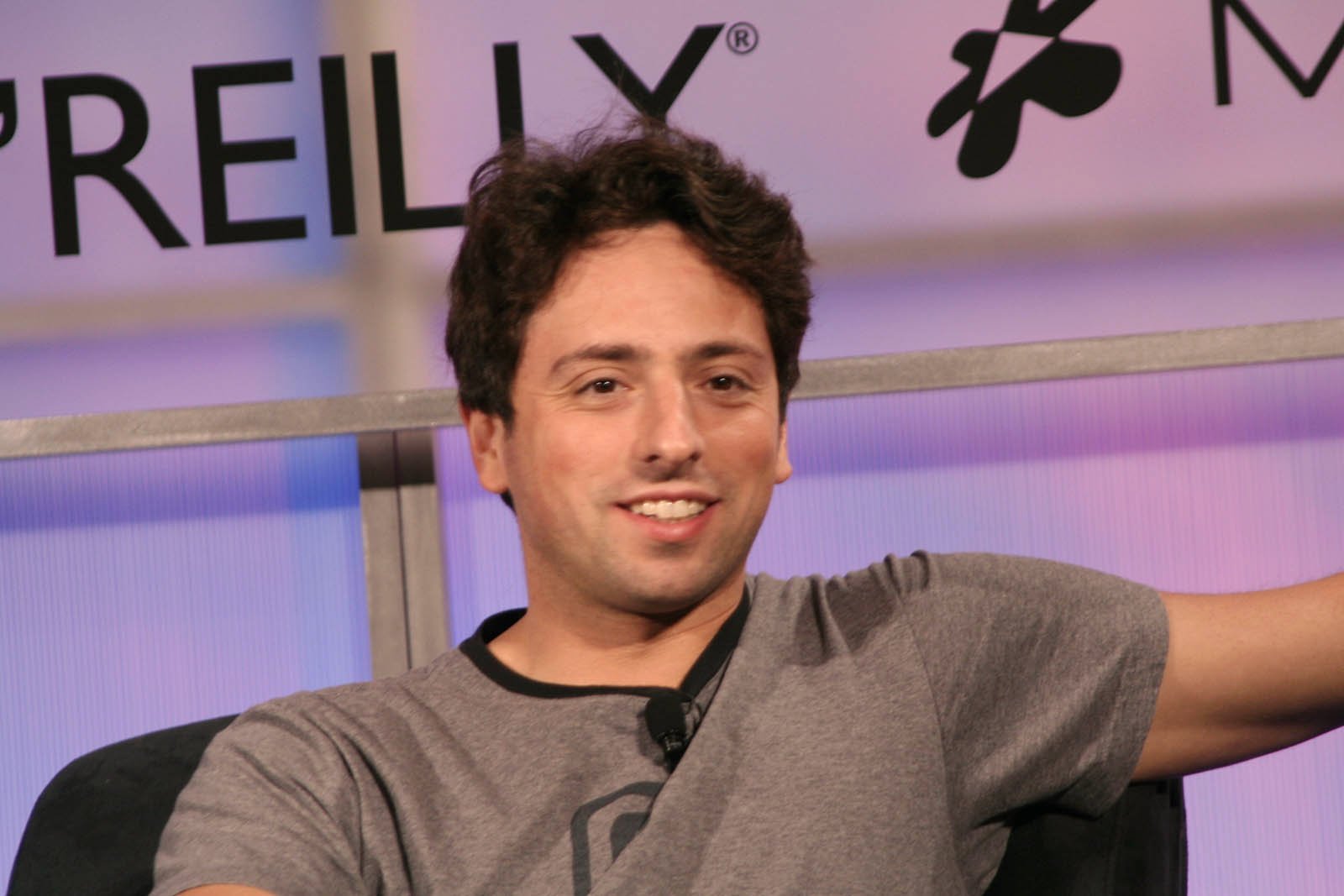In the image, there is a man resembling Sergey Brin, who appears to be in his early 30s, with medium-length dark, wavy hair and dark brown eyes. He is sitting in a black chair, dressed in a medium to dark gray V-neck t-shirt with a black logo partially obscured, and a small lapel microphone is clipped to his shirt. He is positioned slightly turned to his left, facing just past the camera, and smiling warmly, with wrinkles visible at the corners of his eyes. His left arm is outstretched to the side, revealing part of his underarm. The background features a purple backdrop with wood trim and letters ending in "R-E-I-L-Y" in black, and a logo with a rounded star and triangle in it, as well as another partially obscured letter. The setting suggests he is addressing an audience, possibly during a talk or presentation.